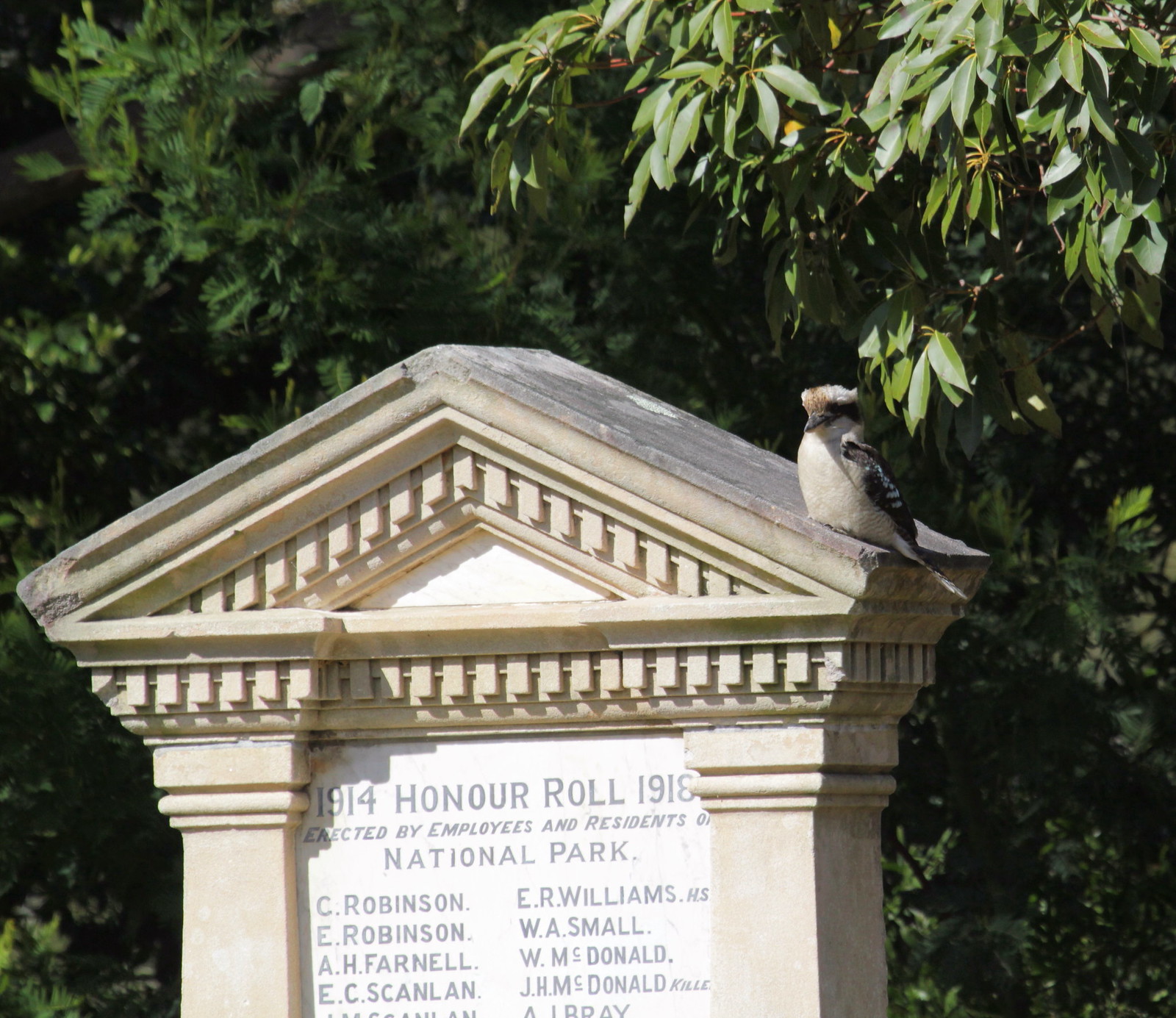This photograph captures a high-quality, 8x8-inch image of a concrete memorial monument with a slanted roof, resembling the architecture of a small structure complete with design elements like pillars. The monument, set against a backdrop of dense shrubs and trees, bears the inscription "1914 Honor Roll 1918. Erected by employees and residents of National Park." Listed on the monument are the names: C. Robinson, E. Robinson, A.H. Farnell, E.C. Scanlon, E.R. Williams, W.A. Small, W. McDonald, and J.H. McDonald, who is notably marked as "Killed." Perched atop the right side of the monument's roof is a small, brown and white bird, possibly a laughing kookaburra. While the foliage in the background hints at a wooded area, the tops of the trees and the skyline are not visible in the image.